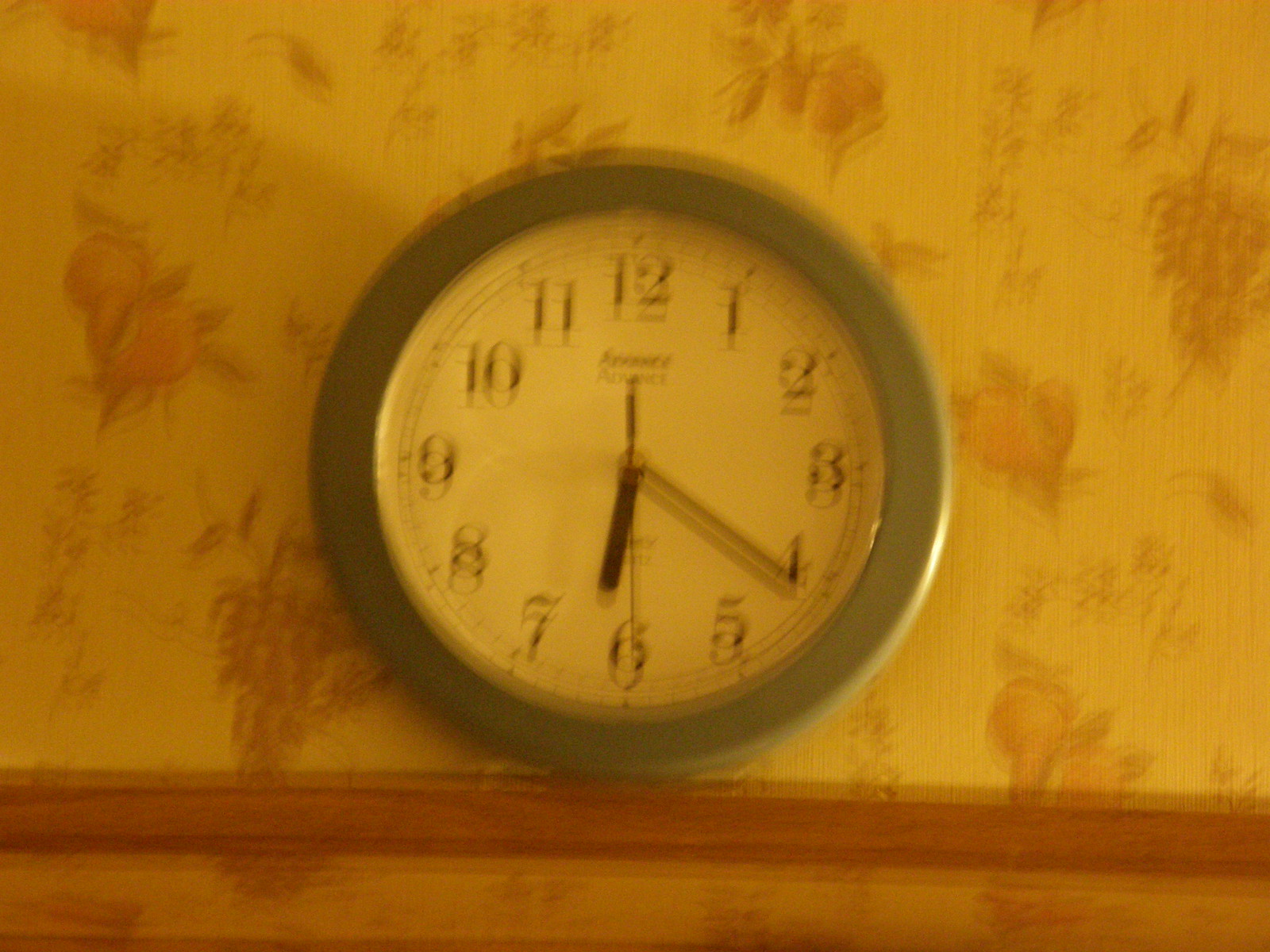The image, though slightly blurry, captures a section of a wall adorned with vintage wallpaper featuring bunches of grapes and possibly other fruits, like pears. At the upper portion of the frame, part of a door frame is visible beneath the wallpaper. On the small ledge nearby, there's a round wall clock prominently displayed. The clock has a green-trimmed frame, and its face clearly shows all the numbers from 12 to 11. The time indicated on the clock is approximately 6:22, with a visible second hand in addition to the hour and minute hands.